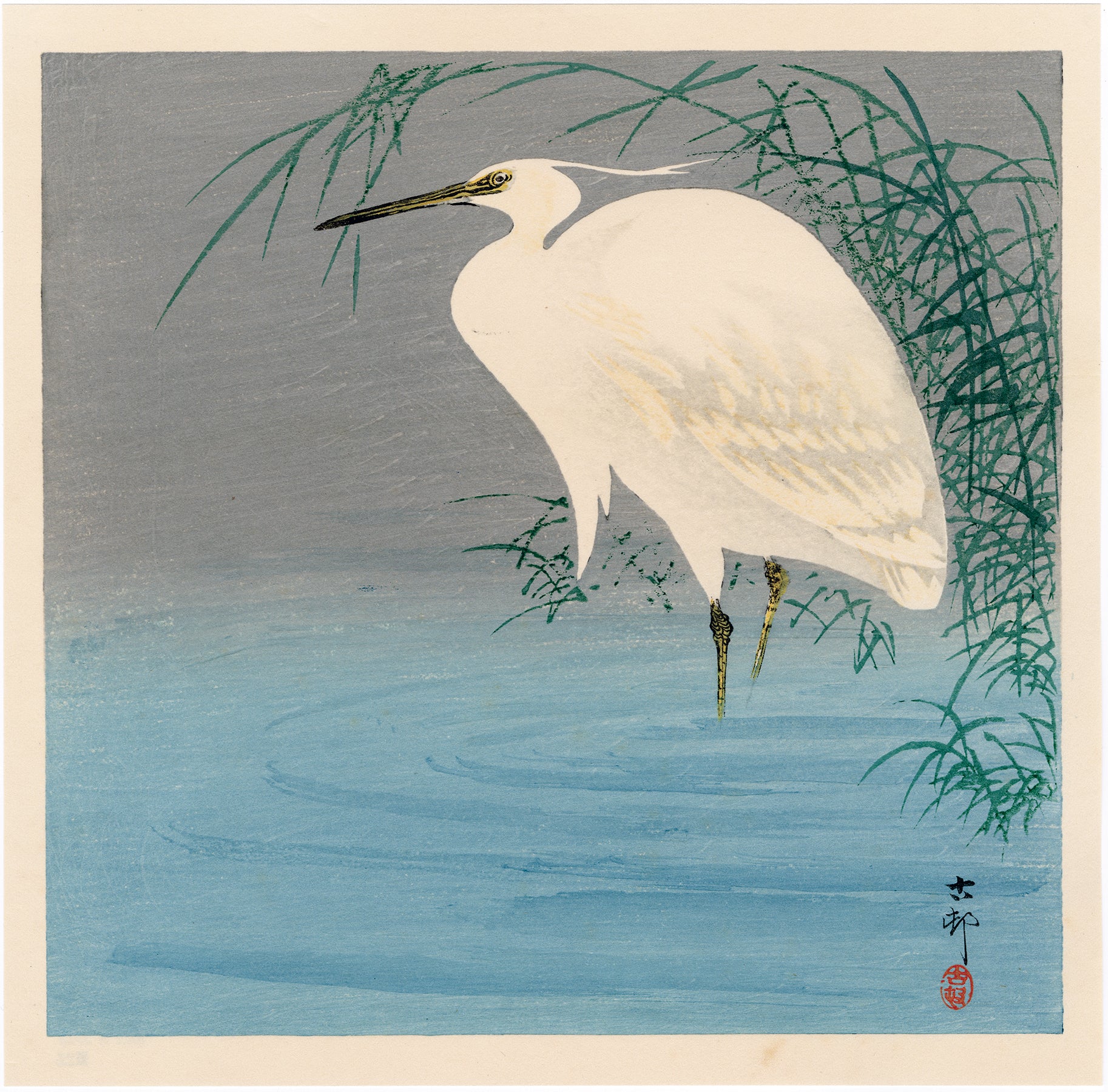This image showcases an antique-style Japanese painting, rendered on faded beige paper. The focal point is a prominent white crane, characterized by its long, slender yellow beak and light black eyes. The crane, facing left, stands in a pool of light blue water, its thin yellow legs partially submerged, rendering its feet invisible. The bird's head, adorned with a feather that swoops out behind it, is relatively small compared to its large, graceful body.

Surrounding the crane are green, wispy grasses with long stems, which appear to be either bamboo shoots or other aquatic plants rising from the water, contributing to the serene ambiance. The background transitions from the light blue water to a gray expanse further in the distance, enhancing the depth of the scene.

In the lower right-hand corner of the painting is the artist's signature in black Japanese characters, accompanied by red text below it. This signature adds an authentic touch to the vintage aesthetic of the artwork. The painting is either framed in a cream color or bordered by paper, enhancing its antique appearance.